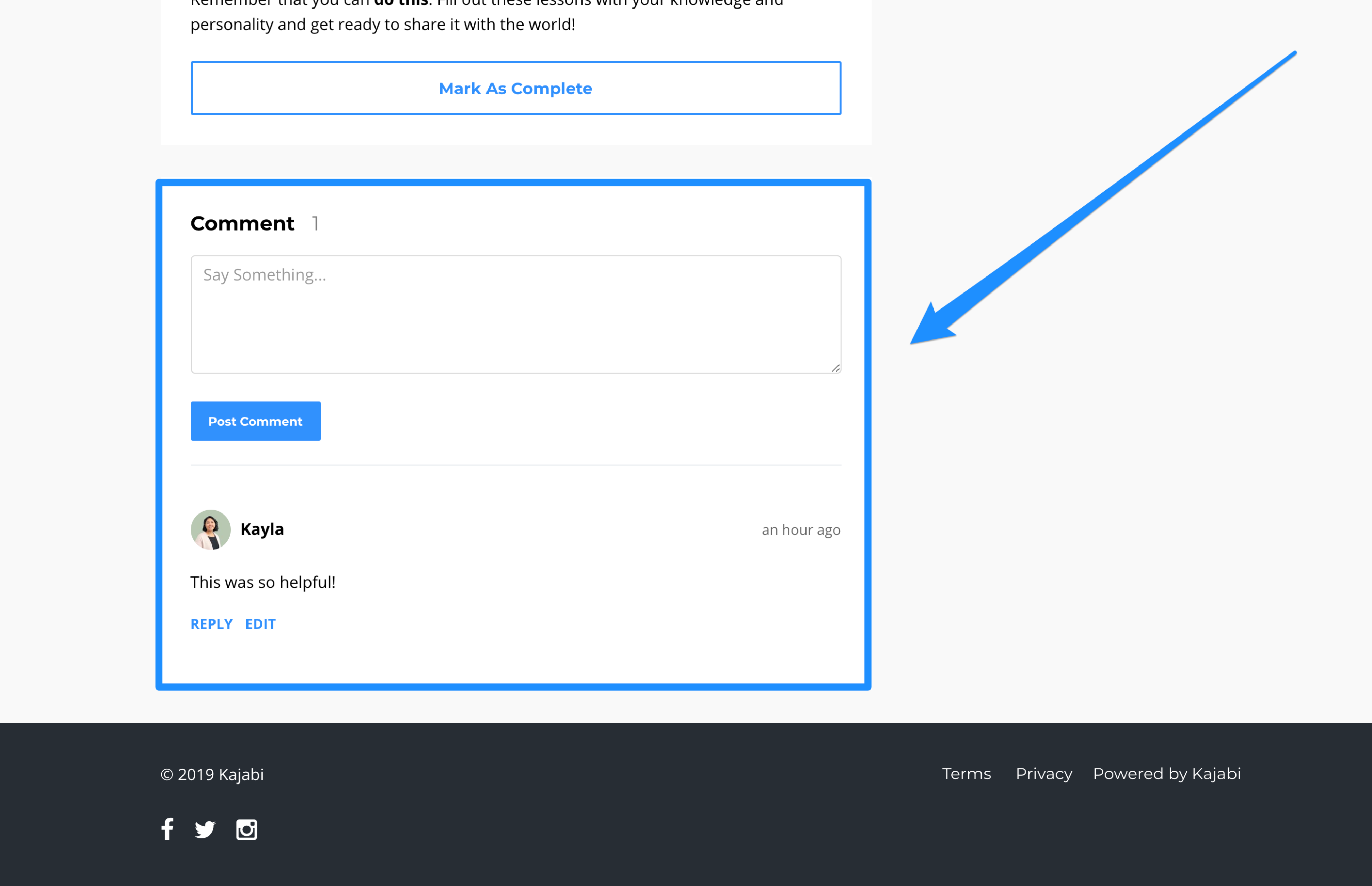In this image, we see a detailed screenshot of a computer screen displaying a section of a website. At the top, the page has a prominent message that reads, "Personality and get ready to share it with the world!" in bold text with an exclamation mark for emphasis. Just beneath this message, there's a white rectangular button outlined in blue that states, "Mark as complete."

Further down, we encounter a white square with the label "Comment" in black text accompanied by the number "1." Below this, there is another white rectangular area with a light gray text prompt that says, "Say something..." indicating a text input box. Adjacent to this input area is a button labeled "Post Comment" in white text on a blue rectangular background.

Moving below this section, a profile picture of a woman appears. She is dressed in a white sweater layered over a black blouse. The name "Kayla" is displayed in black text with a capital "K." To the right of her name, it notes that she posted her comment an hour ago. Kayla's comment, in black text, enthusiastically states, "This was so helpful!" followed by an exclamation mark. Beneath her comment, there are two action options in blue, uppercase letters: "REPLY" and "EDIT."

At the bottom of the screen, the footer displays the text "© 2019 Kajabi," along with icons for Facebook, Twitter (now rebranded as X), and Instagram. To the right, there are links labeled "Terms," "Privacy," and "Powered by Kajabi."